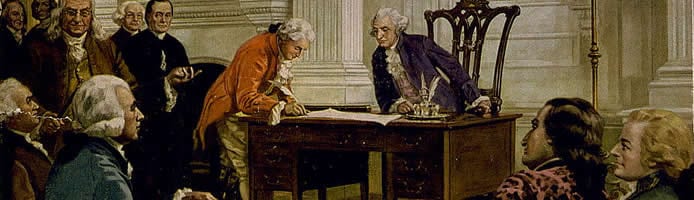The image appears to be a well-lit, highly detailed oil painting set in a neoclassical style room with white walls, columns, and arches. At the center, a man with a light complexion, wearing a rust-colored coat and tan pants, stands next to a desk, signing a large document, likely the Declaration of Independence. The prominent figure behind the desk, bending forward to observe the signing, is dressed in a royal purple coat with white ruffled accoutrement and is reminiscent of George Washington. To the left, another notable figure, Benjamin Franklin, in a brown coat, golden shirt, and white ruffled collar, watches closely. The room is filled with several other individuals, most of whom have gray hair or are wearing powdered wigs, all focused on the central act of signing the document. There are no words or numbers shown in this vividly colorful and clear image, which captures the historical essence and significant gathering for this monumental event.